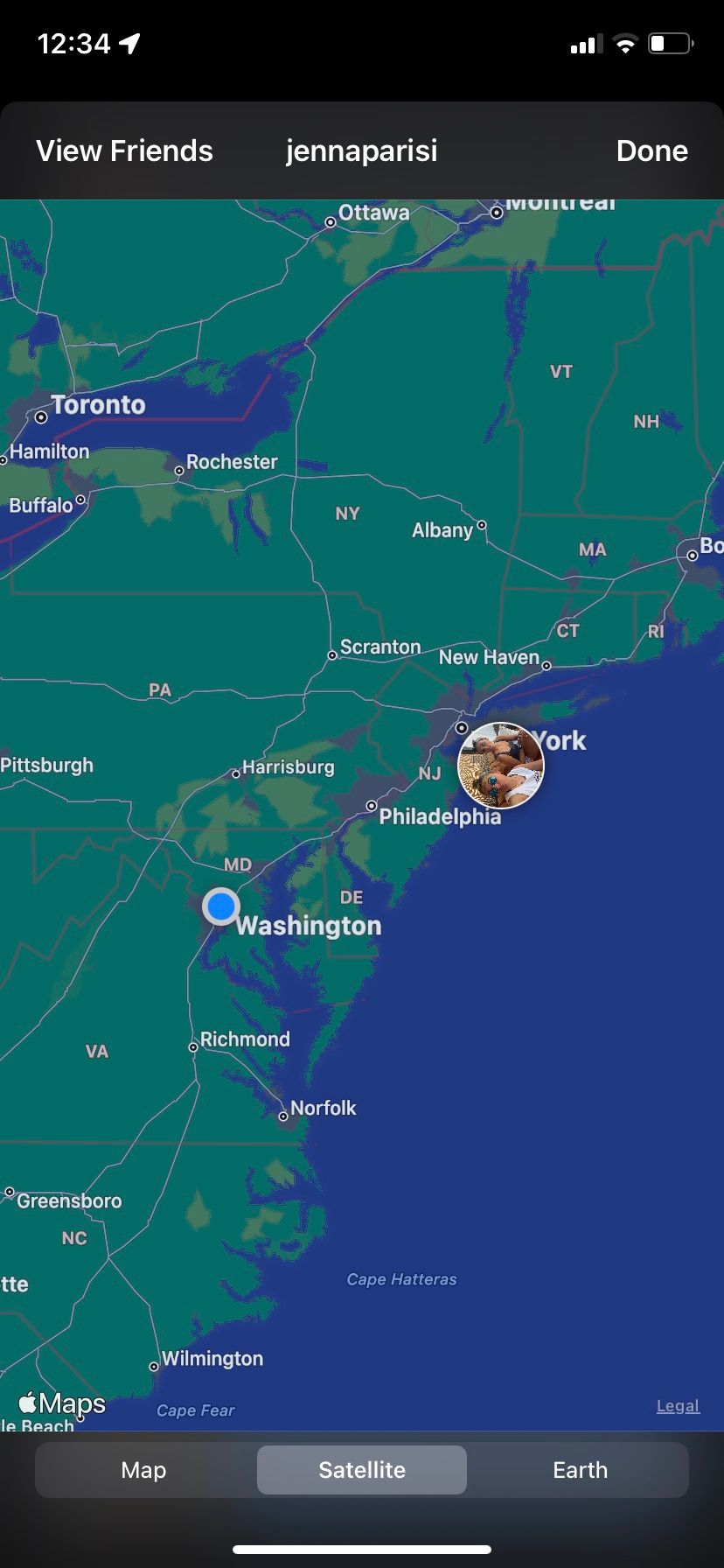A screenshot of a smartphone displays various elements at the top of the screen. The status bar shows the time as 12:34, along with signal strength indicators where the first three bars are white and the fourth one is blank. The battery icon next to it is partially filled in white. Below the status bar is a gray navigation bar with the text "View Friends" on the left, "Jenna Paracy" in the center, and "Done" on the right.

The main section of the screen features a map. The map shows a green landmass and a substantial water region in the bottom right. The map primarily illustrates areas in Canada and the northeastern United States. Key locations labeled include Toronto in the upper left and Ottawa towards the top center. A blue dot marked "Washington" is located in the middle of the screen, although this corresponds to the Washington, D.C. area rather than a city in Canada. A circular avatar is positioned around the New York area, indicating the person's picture. The top part of the map includes Canadian territories, while the right side spans areas of New York and Philadelphia.